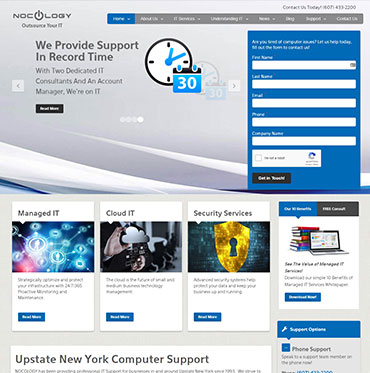The image depicts an advertisement for NOCLOGY, a tech support service specializing in Managed IT, Cloud IT, and Security Services. The central focus is a square box containing their slogan, "We provide support in record time," accompanied by a small clock icon displaying "30," likely indicating the speed of their service. Below this, text states that support is handled by two dedicated IT consultants and an account manager.

On the right side near the top, there's a blue box housing smaller white boxes, possibly for obtaining a service quote or creating a login, though the text is quite small and difficult to read. Below this, a section with a laptop icon and an array of books signifies additional information.

At the very bottom, a white box with black text reads "Upstate New York Computer Support," followed by more text that is too small to discern clearly. The overall theme suggests a professional IT support service tailored to meet various technological needs.